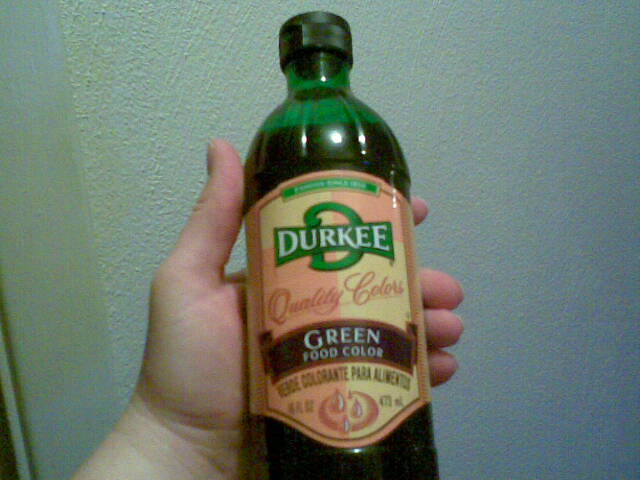This photograph features a light-skinned Caucasian person's left hand prominently positioned in the middle, holding a large, dark green, somewhat transparent bottle filled with liquid up to the top. The bottle, which has a black twist cap, is resting in the open palm of their hand, with the thumb visible on the side. The setting includes a coarse, textured wall in the background, bluish-green in color with a yellowish-brown stain near the left-center. The label on the bottle is peach and pale yellow, with a green trim. At the top of the label, there is a large green 'D' behind a smaller green banner that says "DURKEE" in white letters. Beneath this, in cursive, it is written "QUALITY COLORS," followed by a dark brown banner with white letters that read "GREEN FOOD COLOR." The label also includes the Spanish translation "VERDE COLORANTE PARA ALIMENTOS" and various symbols resembling droplets at the bottom. The overall quality of the photo is not very clear.